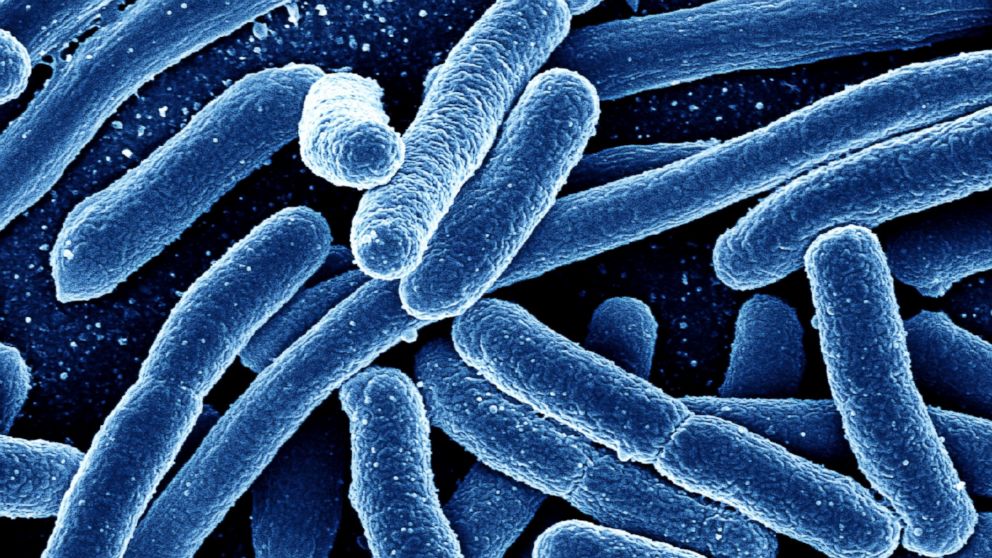This detailed electron microscope image reveals a cluster of bacteria with a striking blue hue, accented by white highlights. The bacteria, which exhibit a sausage-like, or 'wormy' appearance, are intricately stacked and intersecting, varying in length with some spanning nearly the full width of the image. Against a sparkly, dark blue background interspersed with white specks, these microorganisms create a dynamic scene reminiscent of floating blue cheesies. The composition, with its range of blues from very light to almost black, gives an almost artistic quality to the close-up view of around twenty bacteria, each distinct yet part of the intricate biological tapestry.